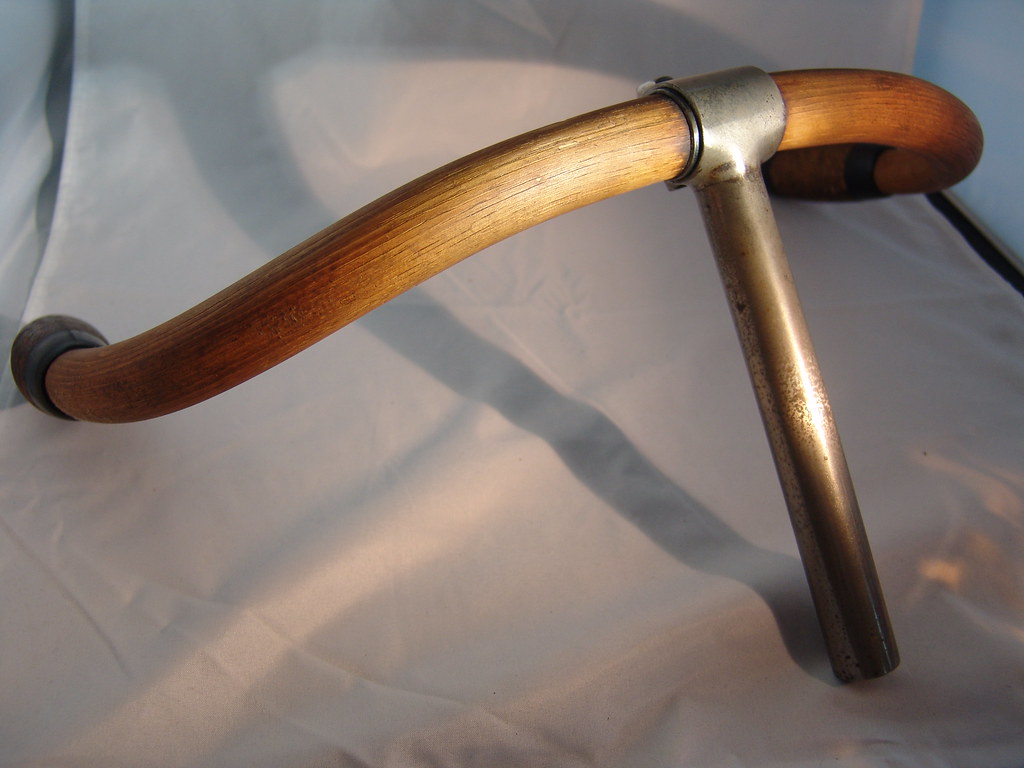The image showcases a vintage wooden and metal object resembling the handlebars of an old bicycle. The handlebars are crafted from curved brown wood, accented with black plastic coverings on both ends, which appear soft like grips. The wood features visible brown streaks, adding to its antiquated charm. At the center of the wooden handlebar, a somewhat rusty metal bar is secured, suggesting its possible use as bicycle handlebars in the past. The entire assembly rests upon a white, slightly rippled cloth, which is gently illuminated by warm, soft sunlight from an unseen source, adding a nostalgic touch to the scene.